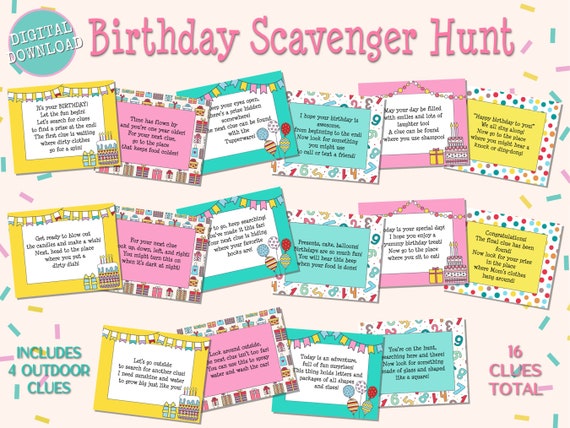This image is a digital download flyer for a 'Birthday Scavenger Hunt,' characterized by a festive and colorful design. The backdrop is an olive hue, with a light blue circle at the top left corner labeled "digital download" in white text. Prominently displayed in large, darker pink letters to the right is the title "Birthday Scavenger Hunt." The flyer features a cascading illustration of confetti in pink, green, and yellow hues along the left and right borders, evoking a celebratory mood.

At the center of the flyer, there are three rows of vibrant clue cards, each intricately designed with various colors and borders: yellow, pink, and blue. These cards alternate between these colors and house different clue poems and decorations, such as banners, numbers, and birthday cakes. The writing on each card may be challenging to read, adding an element of mystery to the scavenger hunt.

In the bottom left corner, the flyer notes "includes four outdoor clues," while the bottom right confirms "16 clues total," highlighting the comprehensive nature of the scavenger hunt experience. The overall design, laden with detailed illustrations and colorful elements, promises an engaging and entertaining activity for birthday celebrations.